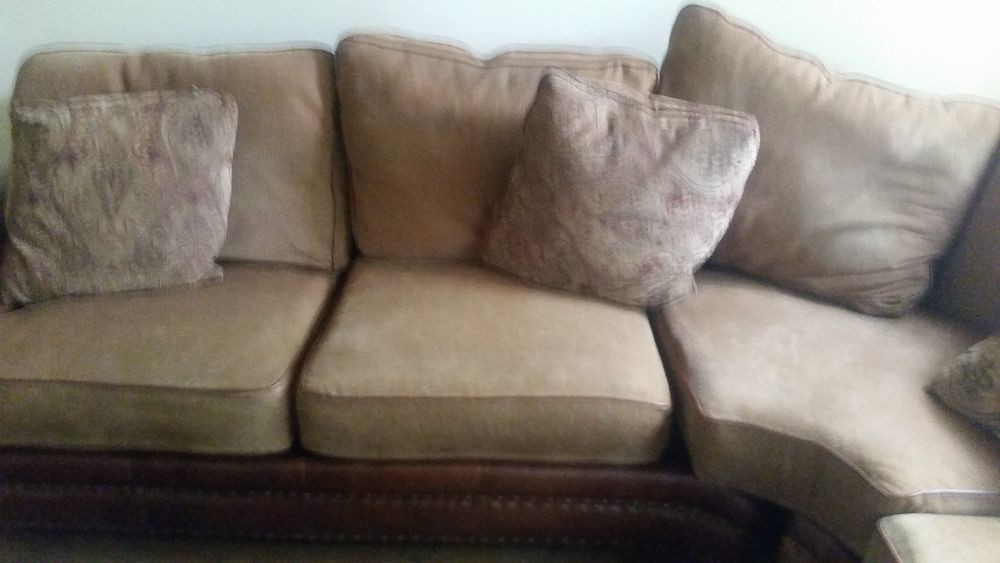This photograph, though slightly blurry, captures a sectional couch situated in a household. It prominently features a corner section with the front and corner cushions extending toward the bottom right of the frame, though the full length of the sectional is not visible. The couch is upholstered in light brown leather, which contrasts with the darker brown leather base. The leather upholstery presents a visible texture across the cushions, pillows, and base. Notably, the base also showcases detailing that resembles small ornamental beads, adding a touch of elegance.

The sectional is designed with large squared cushions that transition into a rounded corner piece, creating an L-shape typical of such couches. This rounded corner has a unique trapezoidal form that facilitates a 90-degree angle. The couch cushions, comfortable and tan-colored, are slightly misaligned at the back, creating a lived-in look. Adding to the decor are throw pillows featuring a maroon-hued design, with two fully visible and a corner of a third peeking into the frame. The entire couch rests on a scalloped wooden frame, enhancing its stylish appearance and comfort.